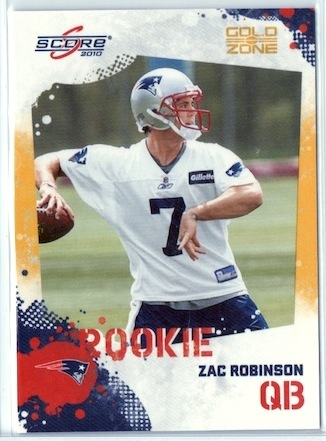This image features a rookie card for Zach Robinson, the quarterback for the New England Patriots, evidenced by the emblems on his uniform. The card has the "SCORE 2010" emblem in the upper left-hand corner and the "GOLD ZONE" emblem in the upper right-hand corner. At the center of the card, a photograph captures Zach Robinson mid-throw, wearing a Patriots helmet while seemingly at practice, as he is not fully geared up. Beneath the photo, the word "ROOKIE" is prominently displayed, indicating that this is his first-year card. Below "ROOKIE," on the lower right, his name, "Zach Robinson," is printed along with his position, "QB." The card design is detailed, making it a significant collectible item for fans.